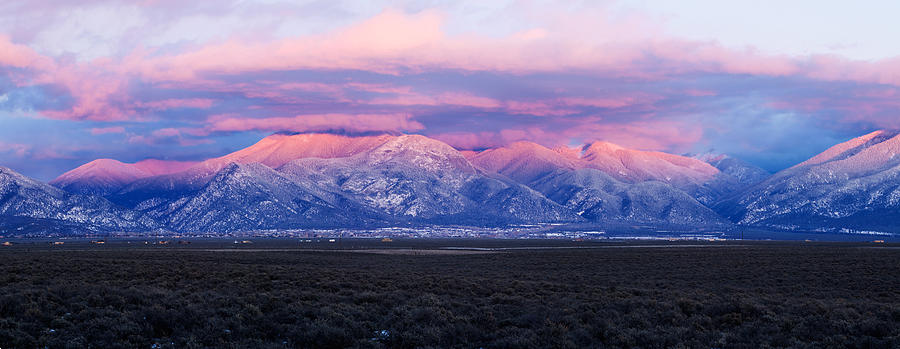A stunning wide-angle photograph captures a vast and serene mountain landscape. The foreground features a broad tundra-like field with indistinct flora and a hint of water right at the base of the mountains. The distance reveals an extensive range of majestic, snow-peaked mountains, cloaked in a breathtaking palette of pastel grays, pinks, and blues, evocative of a sunset or near-sunset scene. The towering peaks, adorned with a dazzling mix of purplish-pink and light blue from the setting sun, are sharply defined, suggesting the use of a high-quality camera by the photographer positioned 10 to 20 miles away. Above the mountains, the sky is filled with striated lenticular clouds blending hues of pink, gray, and dark to light blue, adding to the tranquil beauty of the scene. The image also subtly hints at a town nestled at the foot of the mountains, enhancing the picturesque and serene qualities of this striking landscape shot.